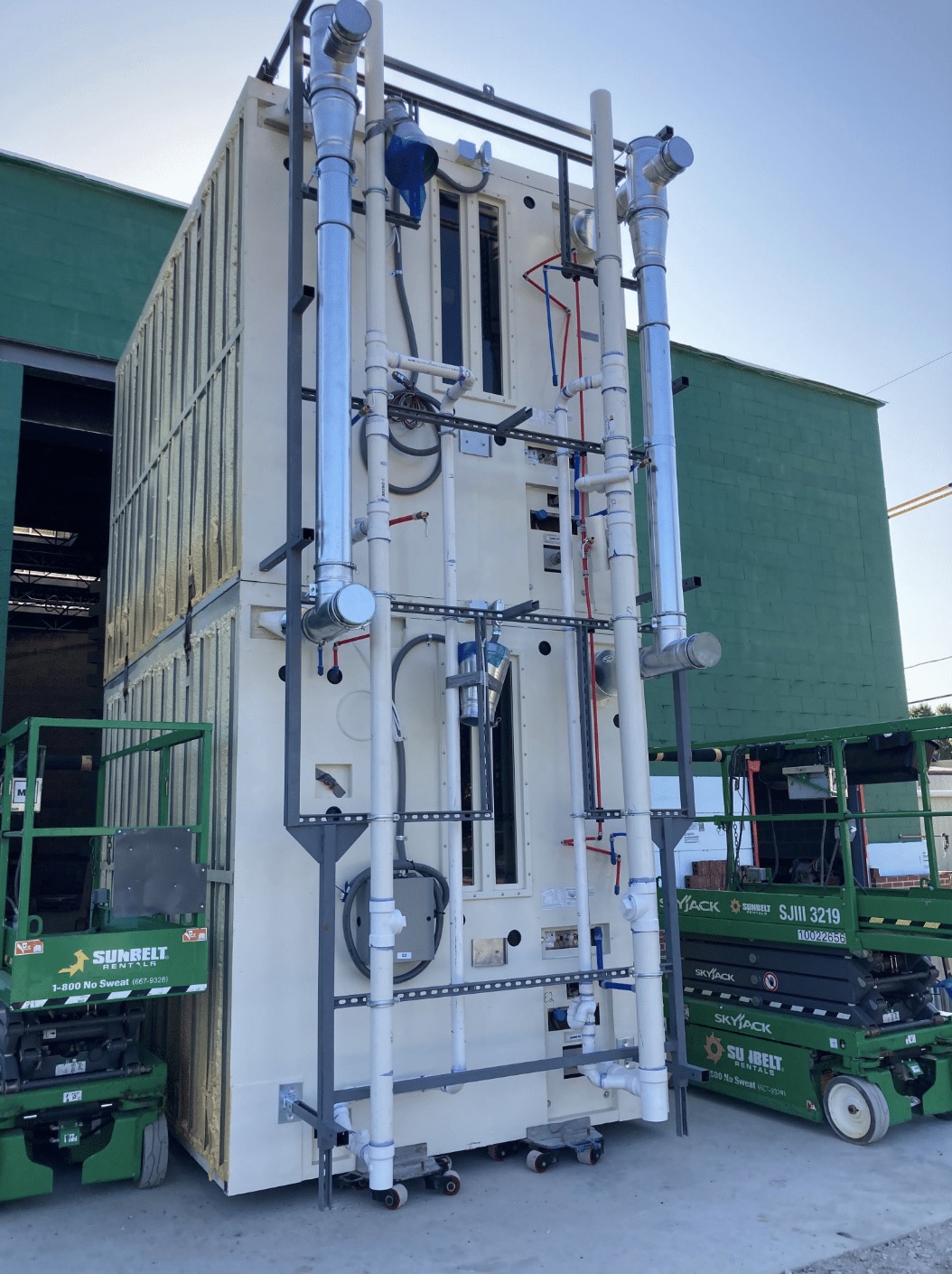The image depicts an industrial area featuring a large, beige two-story piece of equipment with a towering, rectangular shape and flat sides. Dominating the middle, this massive structure is adorned with various interconnected components, including numerous pipes in bone white and silver, red wiring, and blue piping. Vertical white slats and gray metal bracing, along with horizontal support beams, reinforce its robust frame. The equipment appears somewhat like a giant dumpster or storage crate, accentuated by metal braces and brackets.

Flanking this centerpiece are two green and gray scissor lifts, each equipped with platforms and wheels, designed for workers to reach the equipment’s upper sections. The scene is set against a backdrop featuring a large hanger-type building with a significant overhanging opening on the left, revealing a darkened interior illuminated by overhead lights. Adjacent to this building is a brick-faced structure painted in forest green. Above, the sky is a light blue, providing a stark contrast to the industrial elements below. The ground is cemented, suggesting a warehouse-style environment, likely utilized for heavy maintenance or storage.